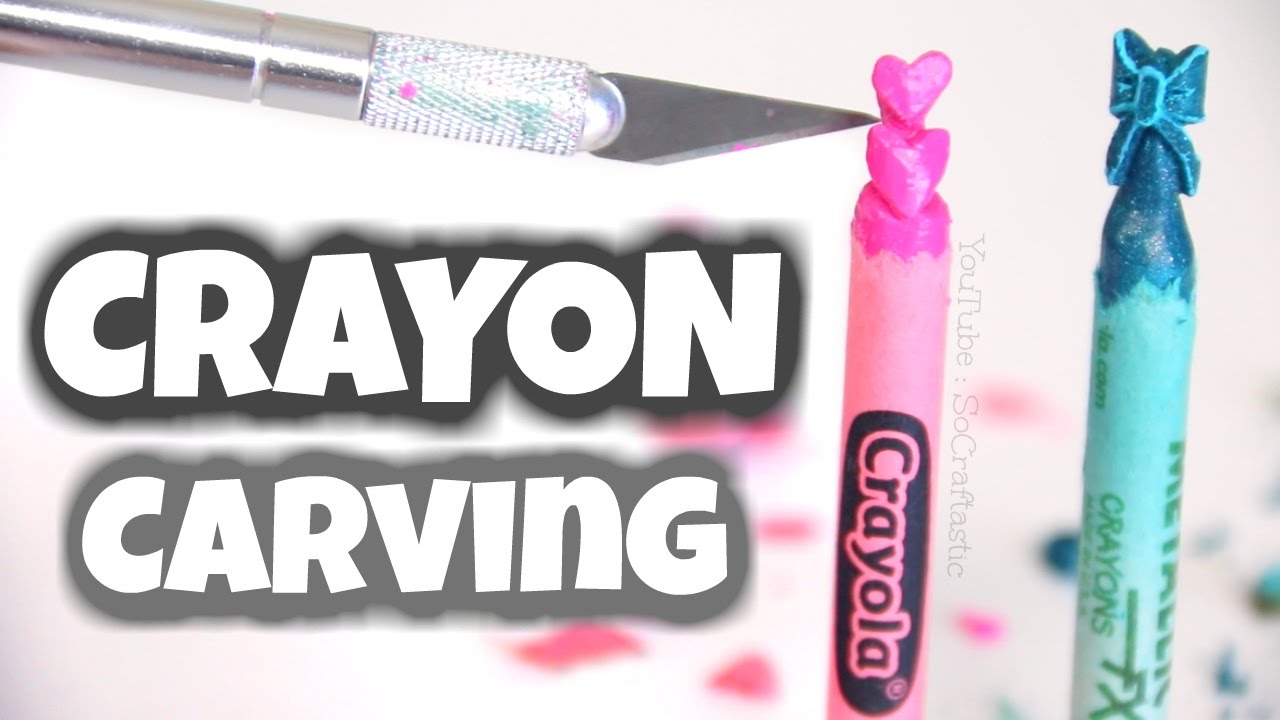The image poster, titled "Crayon Carving," showcases a detailed demonstration of intricate crayon art. Set against a grayish-pink background, the large white text with a prominent black drop shadow spells out "crayon carving," with "carving" appearing slightly more transparent. The focal point of the image is a very sharp, fine-edged scalpel knife that stretches from the left to the right side of the poster, highlighting its precision by having its tip delicately touch the edge of a pink crayon. The pink Crayola crayon, positioned vertically, has its tip meticulously carved into the shape of two hearts. Beside it, a blue (or teal) Crayola crayon displays its tip skillfully transformed into a bow tie. Both crayons have had their paper slightly peeled back, revealing semi-intricate carvings. Flecks of pink and blue are scattered in the background, adding to the artistic theme.